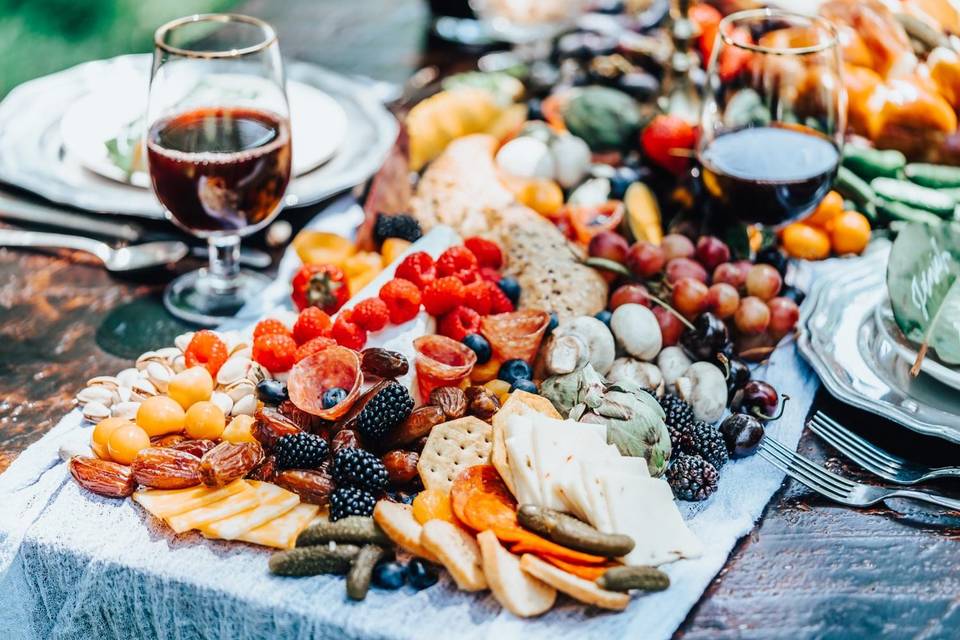The image depicts a vibrant and elaborate charcuterie board placed on a table, which is the main focus amid a slightly blurred background. This board is artfully arranged with a plethora of items, including a variety of cheeses like Colby Jack, Swiss, and Pepper Jack. It also features an assortment of fruits such as raspberries, blueberries, blackberries, and grapes, along with other elements like pickles, mushrooms, and almonds. Pepperoni slices, some formed into cones, are scattered among several types of crackers and nuts, including pistachios. Accompanying the charcuterie board are two half-filled wine glasses, flanking a blue plate adorned with a leaf that bears a signature, suggesting artistic detail in the presentation. Additionally, two forks are positioned next to the plate, and some green vegetables and other foods are visible but blurred in the background, providing a contrast to the sharply focused charcuterie board.